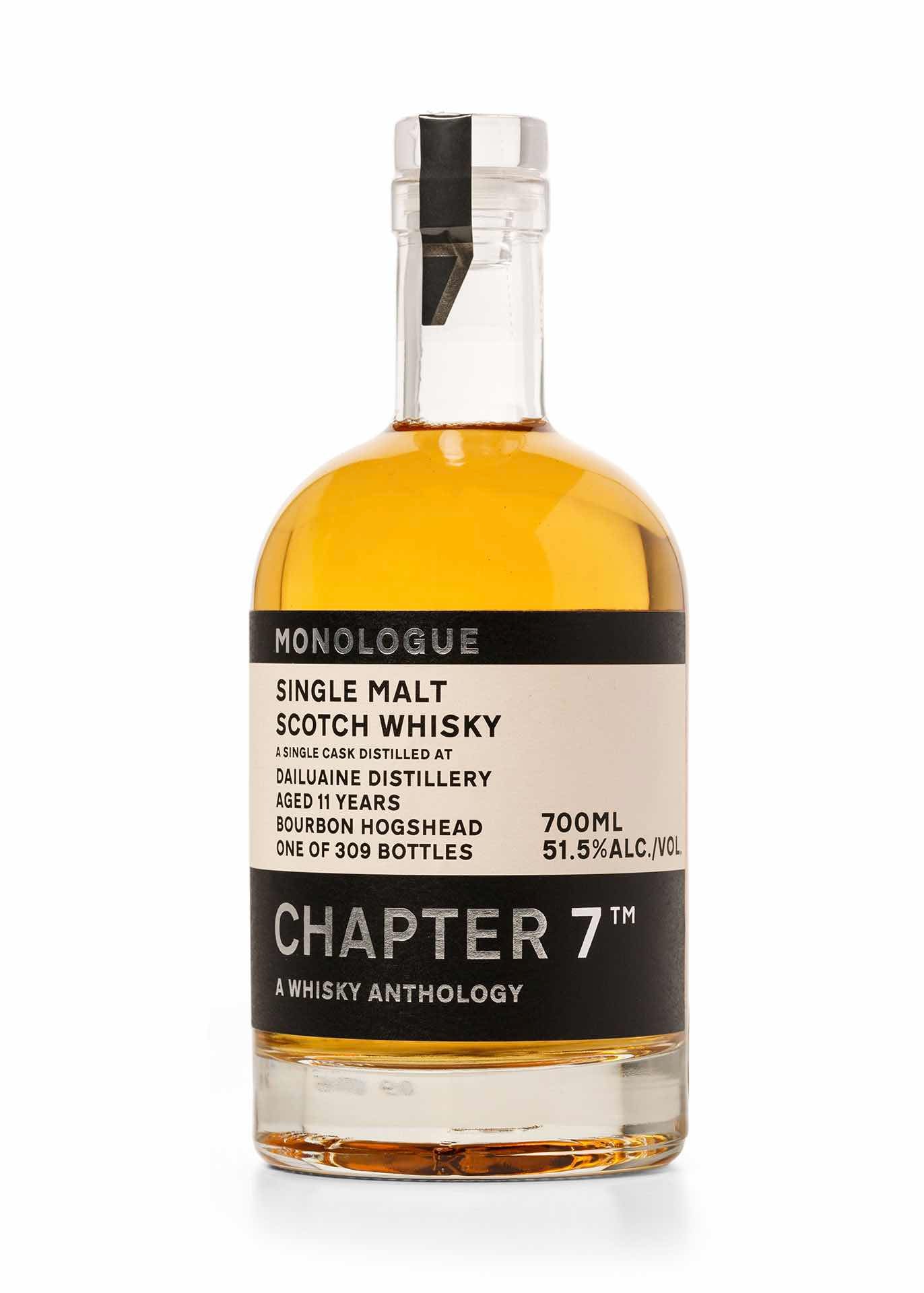This image features a front-facing bottle of whiskey set against a transparent white background, casting a subtle shadow or reflection at the base. The bottle is clear, both the body and the neck, with a distinct clear cap. A black tab or tape runs halfway down the neck, which then extends into a more bulbous main portion filled with amber-yellow liquor.

The whiskey bottle has a detailed label approximately split between a black and a beige (white) section. At the top of the label, within the black strip, the word "Monologue" is prominently displayed in silver. Below this, the beige portion of the label features black text detailing the contents: "Single Malt Scotch Whiskey, Aged 11 Years, Bourbon Hogshead, One of 309 bottles." Additionally, specifics such as "Distilled at Dailuaine Distilleries," "700 milliliters," and "51.5% Alcohol per Volume" are noted. 

The bottom part of the label is again black, stating "Chapter 7™ - A Whiskey Anthology" in silver lettering, marking this bottle as part of a curated series. The clear and descriptive layers of the label ensure all crucial details about the whiskey are easily visible and readable.